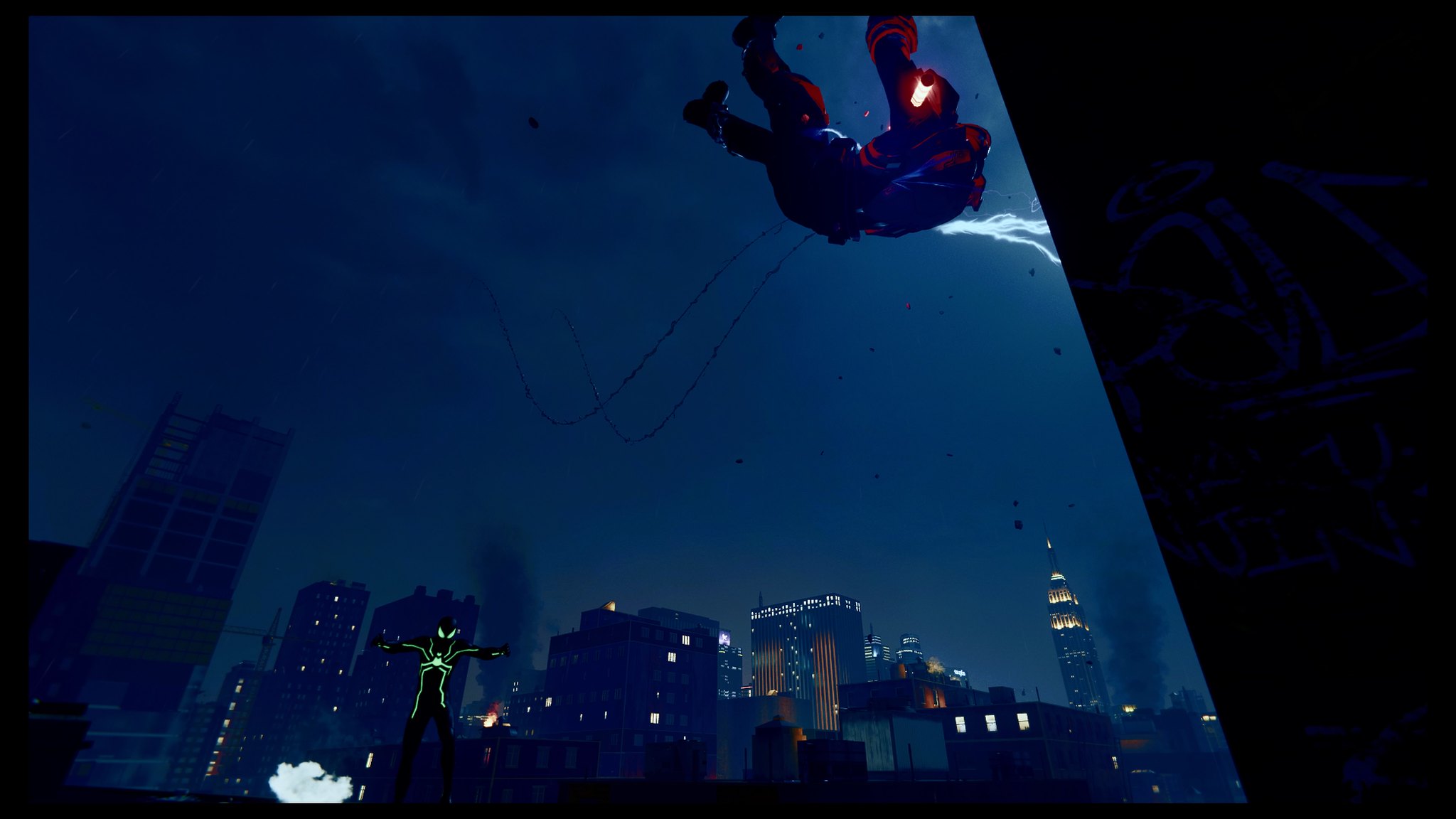In this dynamic image, Spider-Man is captured mid-action as he catapults off a skyscraper, donning his iconic red and blue suit. A red hood with a light attached to the front adds a twist to his traditional look. The cityscape below him, likely New York, is dotted with high-rise buildings including the Empire State Building, grounding the scene in an urban setting. On a nearby rooftop, a figure dressed in a black outfit with green accents on the ears, arms, and body—potentially Catwoman—stands amidst a swirl of white clouds or smoke. The juxtaposition of these two characters against the backdrop of a bustling metropolis creates a vivid and compelling tableau of superhero action and intrigue.